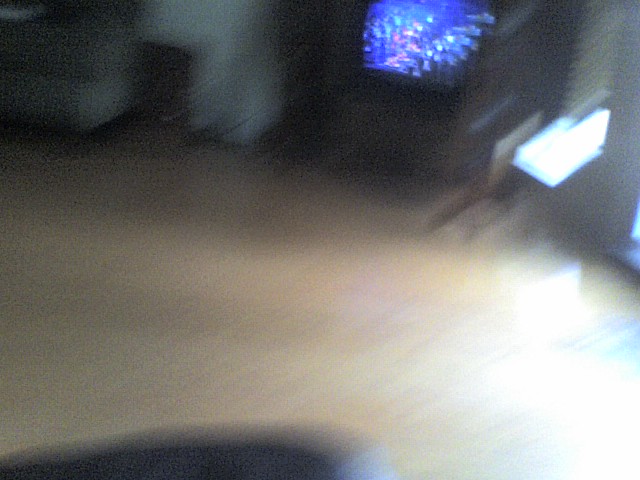The image depicts a slightly blurred scene of a living room, resembling the effect of a camera shake rather than a filter blur. Despite the blur, several elements are discernible. In the background, a gray sofa can be partially seen, likely a full-sized one rather than a chair. Beside the sofa, to its right, appears to be another piece of furniture, possibly a table, although its precise form is difficult to ascertain. Further to the right, a television is visible, encased in an entertainment center. The TV itself seems to be an older model, potentially a CRT unit, which were popular before the 2000s. The screen of the TV shows an array of lights, suggesting the airing of a celebratory or festive program. Natural sunlight filters into the room, illuminating a beige floor that might be either uncovered or carpeted.